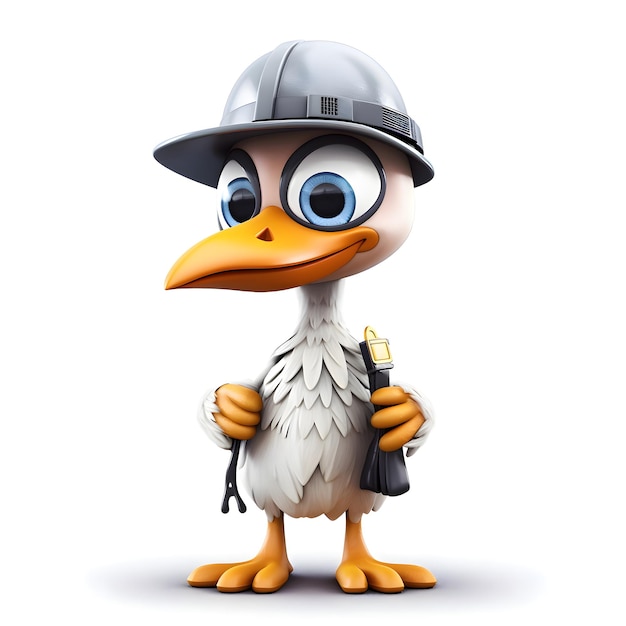This is a detailed cartoon image of a cute working duck set against a plain white background, giving it a clean and simple appearance. The duck is wearing a shiny silver hard hat secured with a strap under its beak, which is large and vividly orange. Its enormous, expressive eyes are beautifully detailed, with black outlines, white accents, blue irises, and black pupils. The duck’s body features textured white feathers, a slender neck, and prominent orange feet with three toes each. In its yellow hands, the duck is holding what seems to be a screwdriver and another indiscernible tool, possibly suggesting it's ready for some construction or factory work. Casting a subtle gray shadow beneath it, the duck appears eager and prepared to tackle any task ahead.